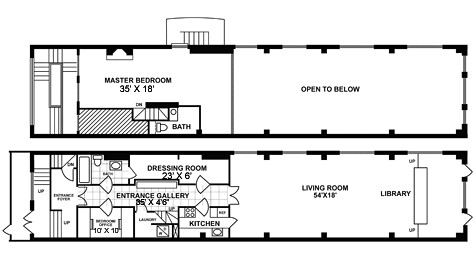This black-and-white diagram is a detailed floor plan consisting of two horizontal sections, one placed above the other. 

In the top portion of the image, on the very left, there is a small section indicating a doorway with some lines. Adjacent to this is a spacious master bedroom measuring 35 by 18 feet. Below the master bedroom, there's an area featuring a stairway and a bathroom. The bathroom, indicated by a toilet symbol and labeled 'bath,' is divided into two sections. 

To the right of this area, a large open space is marked as "open to below," suggesting it may be a double-height space or overlook an area on the floor below.

In the bottom portion of the diagram, to the right, there's a living room measuring 54 by 18 feet. Directly adjacent to the living room is a library, with no separation shown between the two spaces.

The left part of the bottom section includes several rooms. There is a dressing room with dimensions of 23 by 6 feet and an entrance gallery that spans 35 by 4 feet. The kitchen area is detailed with symbols representing a stove and a sink. Nearby, there's a laundry room, marked by a cube with a diagonal line and two dots, likely indicating a washer and dryer. Additionally, there is an office space measuring 10 by 10 feet. The main entrance of the floor plan is located on the left side of the diagram. 

Overall, the floor plan outlines are drawn in dark black, with lighter lines indicating interior openings or possibly windows, providing a clear and structured layout of the spaces.